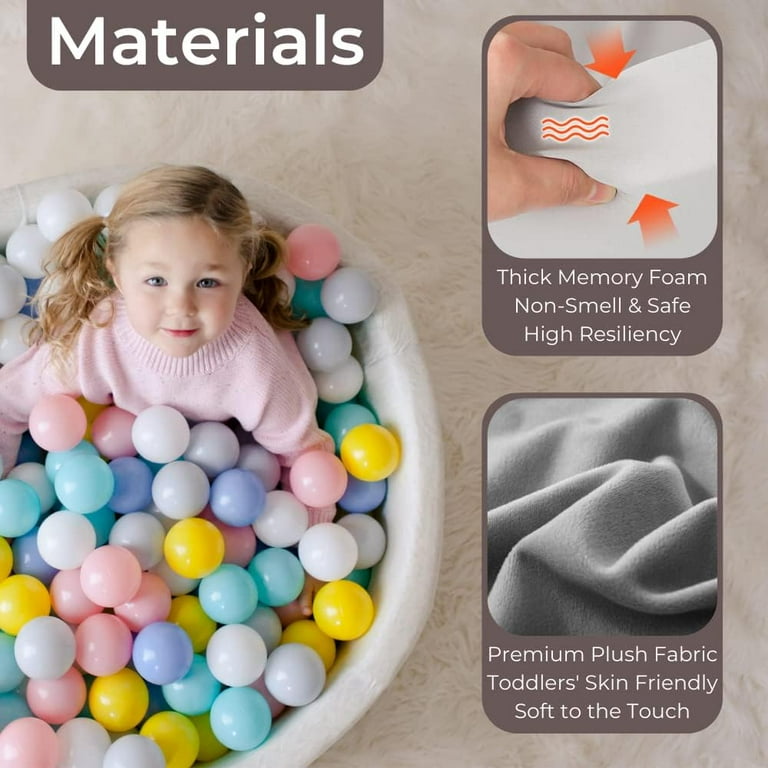The image features a young girl with blonde pigtails wearing a pink sweater, sitting in a colorful ball pit filled with blue, green, yellow, white, and pink balls. The top left corner displays a dark brown bar with white text that reads "Materials." On the right side, there are two separate sections: one shows a close-up of a hand pinching a material with red arrows indicating a thick memory foam that is non-smelling, safe, and highly resilient; the other highlights the folds of a soft, premium plush fabric that is toddler skin-friendly. Behind the girl, there is a blanket draped all around the ball pit. The overall setup emphasizes the safety and comfort features of the materials used in the ball pit.